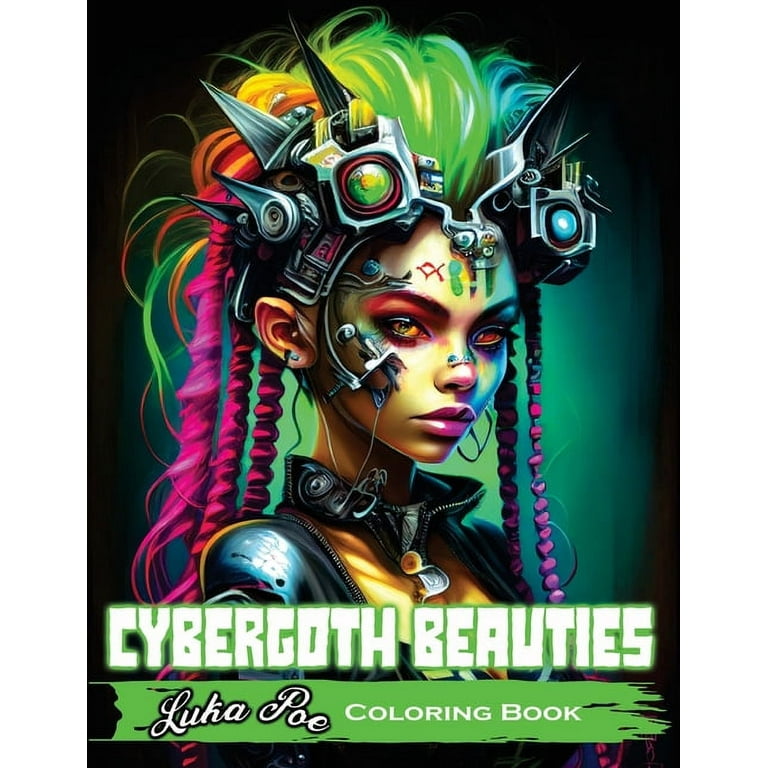The image, seemingly designed or generated by a computer, showcases the vibrant cover of a digital coloring book titled "Cyber Goth Beauties." The central figure is a woman adorned in a striking, zip-up, yellow and black leather suit. She sports an intricate, futuristic headdress with metal-bordered screens—green and blue—with triangular spikes extending outward. Her hair, styled in a voluminous, poofy manner, features a mesmerizing gradient starting with neon green at the top and transitioning into shades of orange, pink, and blue, interspersed with dreadlocks of various colors. Her face is accentuated with colorful and dramatic makeup: smoky black eyeshadow around her yellow and red eyes, red eyeshadow, and pink lips, along with decorative green stripes on her forehead and red lines. She also has a mix of jewelry, including a hoop earring, a piece of gold jewelry on the bridge of her nose, and a metal piece on the side of her face. The background is black, with a transitioning neon green orb behind her, emphasizing her presence. At the bottom, in white text outlined in green, the title "Cyber Goth Beauties" is prominently displayed, with "Luca Poe Coloring Book" noted below in a green banner. This cover fully embodies a futuristic, cyber-goth aesthetic, designed to capture the imagination.